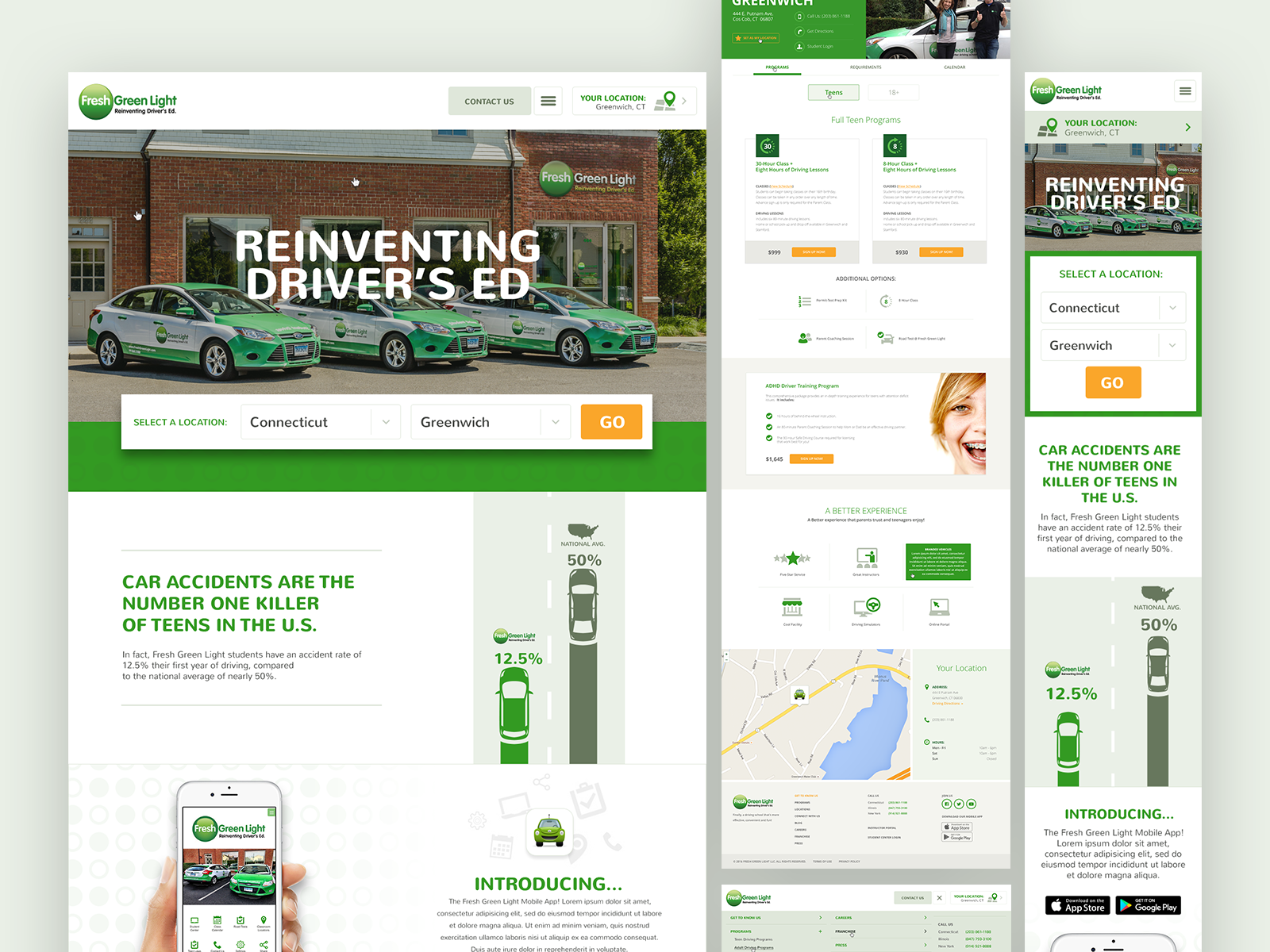The image depicts a car rental page for a company named Fresh Greenlight. The layout consists of three columns, with the first column being the widest and narrowing progressively to the right.

**First Column:**
- At the top, there is a green circle with the word "Fresh" inside it. 
- Positioned next to the circle, "Greenlight" is written in green type, making it clear that the brand name is Fresh Greenlight.
- Below the brand name, there is some text that is not legible.
- To the right of the logo, there is a gray box labeled "Contact Us."
- Underneath, there's a gray rectangle displaying a map with a pin marked in green, indicating the user's location and featuring an arrow pointing right.
- Below the map, in large, bold white letters, there is a statement: "Reinvesting in Drivers Ed." This text overlays an image of three cars that are painted in green and white, all branded with the Greenlight logo. 
- Behind the cars, a brick building is visible, also bearing the Greenlight branding with the words "Fresh Greenlight."

**Additional Details:**
- At the top of the building, a white rectangular box displays "Select Location" in green type.
- Below this box are dropdown menus labeled "Connecticut" and "Greenwich," each with a downward arrow indicating options.
- On the far right end, there's an orange button that has "Go" written in white.

This detailed and structured layout efficiently communicates the brand and services of Fresh Greenlight, emphasizing their investment in driver education and pinpointing user location for convenience.